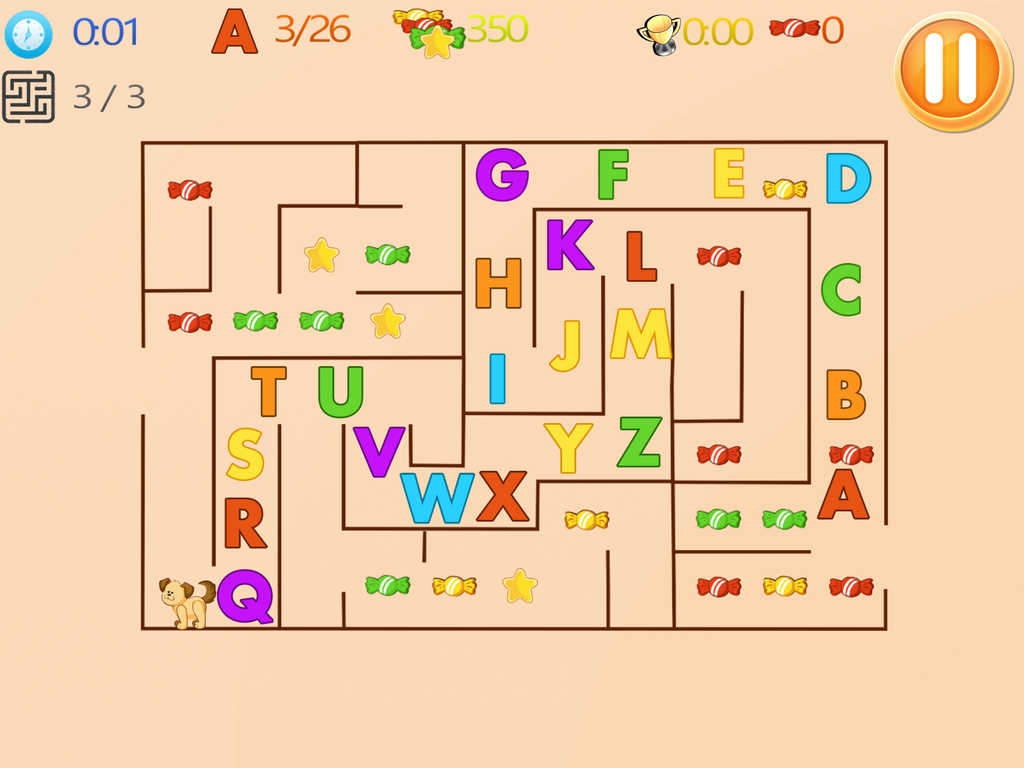The image appears to be a colorful and dynamic game interface from a website. It features a peach-colored background with various interactive elements. In the upper left corner, there's a blue clock icon next to blue text reading "0,01". Adjacent to this is a red capital letter "A" with a red "3/26" next to it. Spread across the image, there are three candies lined up one behind the other: a yellow candy at the back, a red candy in the middle, and a green candy at the front. In front of this trio, there's a gold star followed by green text displaying "350". Across from this arrangement is a gold trophy cup with a yellow "0,00" next to it, and to the right, a red candy with two white stripes marked with a zero. There’s also a gold ring filled with orange, featuring two white lines resembling a paw print.

Beneath the clock, to the left, there’s a black box containing a maze icon, accompanied by the text "3/3" in black. The main section of the image displays a complex maze with a green or black outline, filled with various candies and stars. The left side of the maze prominently features red candies with white stripes, and there are two green candies situated to the right of these. Amongst the candies, gold stars are scattered abundantly. The candies come in red, green, and yellow colors, and the maze is intricately filled with them.

In the bottom left corner of the maze, there's a brown doll characterized by a light brown body and darker brown ears and tails. Scattered randomly across the map are alphabet letters in random order, rendered in vibrant hues of red, orange, green, blue, yellow, purple, and blue. Each letter stands out with its unique color, adding to the vividness of the map.